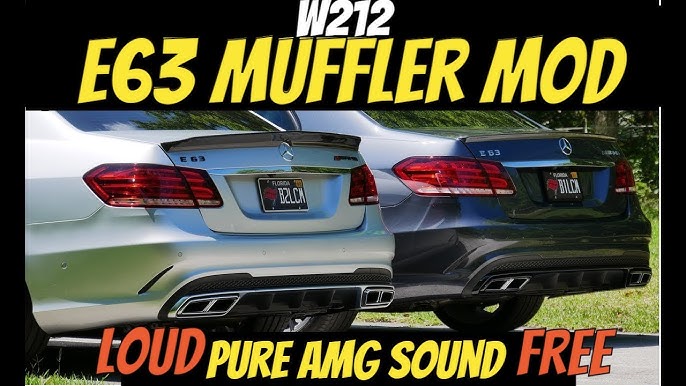The picture resembles a YouTube thumbnail and appears to be an advertisement for a muffler modification. It features a top black banner with "W212" in white text and "E63 Muffler Mod" in large yellow text. Below this, there are the rear ends of two Mercedes-Benz vehicles positioned side-by-side—one silver and one a metallic dark blue or gray—with the Mercedes emblem clearly visible and two dual exhausts on each car. The bottom text reads "Loud Pure AMG Sound Free," with "Loud" and "Free" in orange and "Pure AMG Sound" in yellow. The background displays a green grassy area, and the cars have blue license plates with white lettering, indicating cleanliness and well-maintained condition.